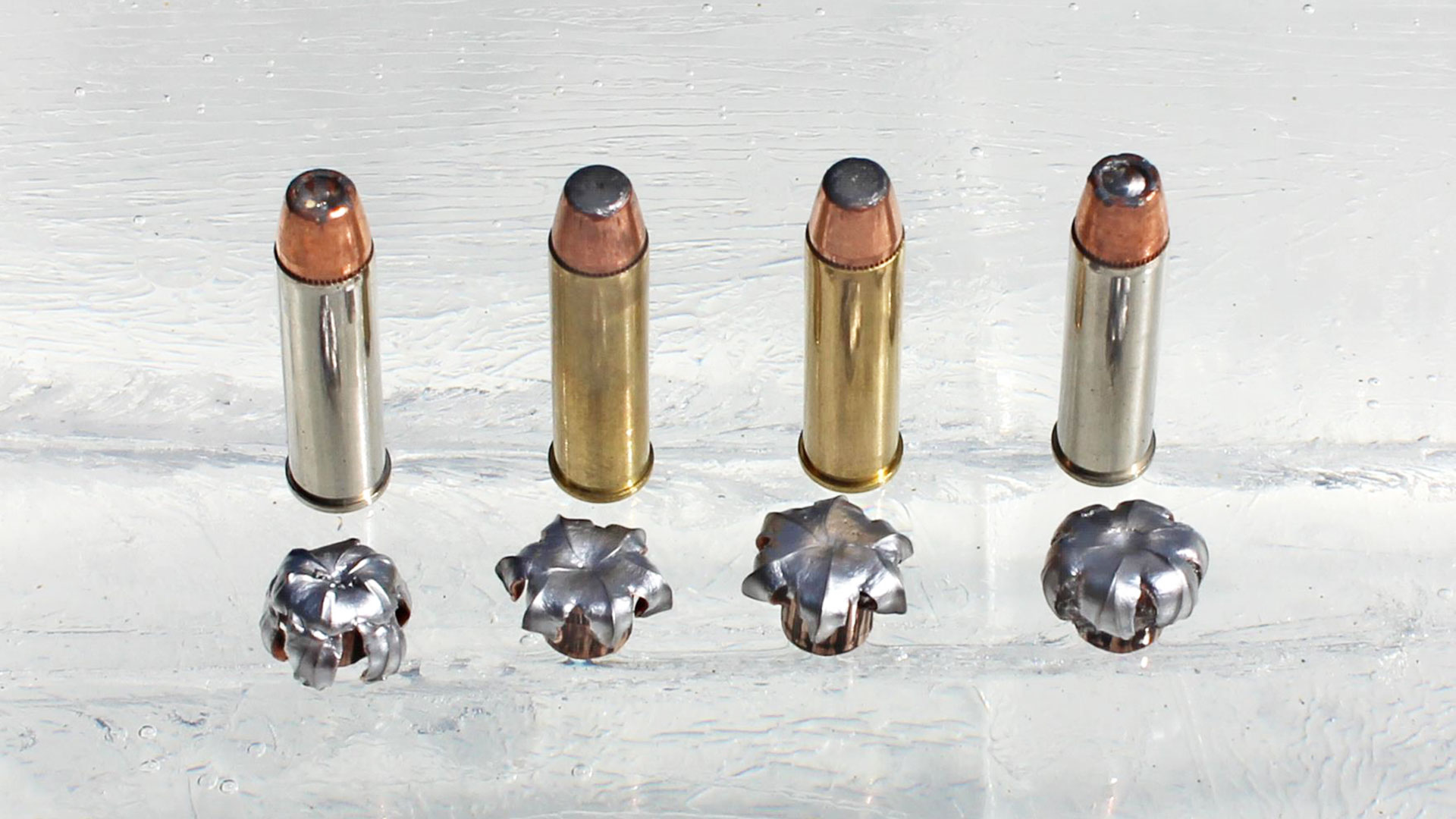The image depicts four bullets, each standing upright and evenly spaced about an inch apart on a frosted glass or marble-like surface. The two bullets in the middle have gold-colored casings with copper-colored tips, while the bullets on the outer edges feature silver casings with copper tips. In front of each bullet lies its counterpart that has been fired and impacted, appearing severely crushed and resembling a flower or star-shaped splat of lead. The overall palette of the image consists of grays, silvers, coppers, and brasses. There is a reflection of windows in the background, suggesting the photo was taken indoors. The surface beneath the bullets is translucent white, adding to the frosty appearance and contributing to the clean, minimalistic setting of the photograph.